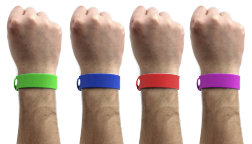This is a detailed photograph featuring four side-by-side wrists, each adorned with a different colored wristband, showcasing the color options for the product. The image, likely a product display, utilizes the same arm presumably edited to illustrate the different colors available. Each wrist is balled into a fist and positioned in a parallel, evenly spaced manner. Starting from the left, the wristbands are neon green, blue, red, and purple respectively. The photograph captures the arms from the fists down to about half of the forearms, and the wristbands appear to be uniform in size and texture. Each band is solid in color with a small silver clasp visible on the left side, emphasizing the variation in color while maintaining the same design.